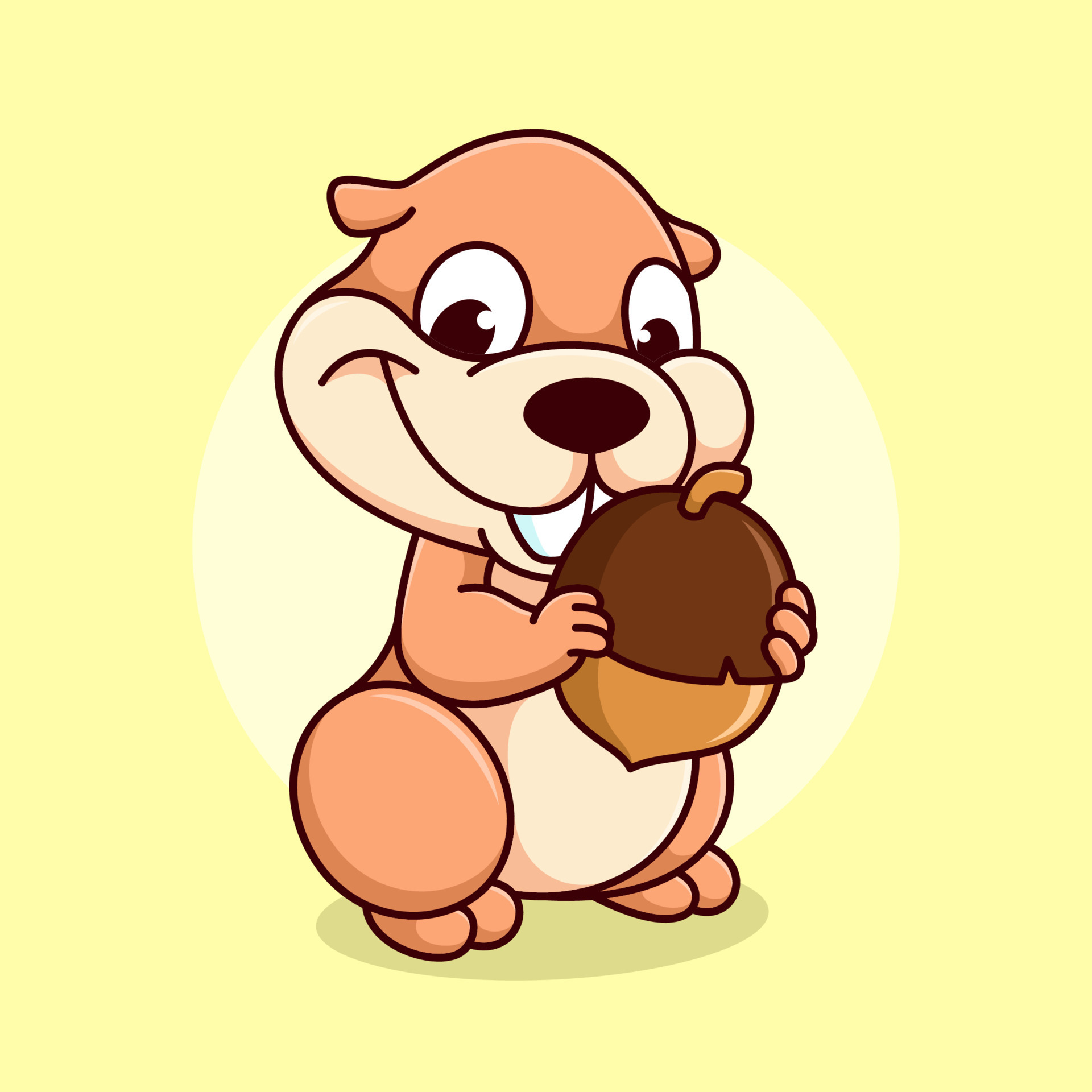This is a detailed cartoon-like drawing of a distinct squirrel-like animal with no tail, featuring over-exaggerated, humorous attributes. The creature is primarily brown with a tan-colored stomach and mouth. Its legs are depicted as large circles, while its toes and bottom paws consist of two round ovals each. The squirrel's head is tan with large, expressive white eyes with black centers, and it has pronounced, protruding white teeth that contribute to its comical appearance. It holds a massive acorn in both hands, gripping it with four fingers. The acorn's bottom is light brown, and its top is dark brown, adding to the visual contrast.

Encircling the squirrel is a light yellow halo, which contrasts with the darker yellow background that fills the rest of the square image. The animal also casts a subtle gray shadow beneath itself, adding a small element of depth. The drawing has all its details outlined in black, giving it a bold, cartoonish look. The overall image resembles an emoji or a computer-generated graphic, with a noticeable smile on the squirrel's face, further enhancing its playful and human-like characteristics.